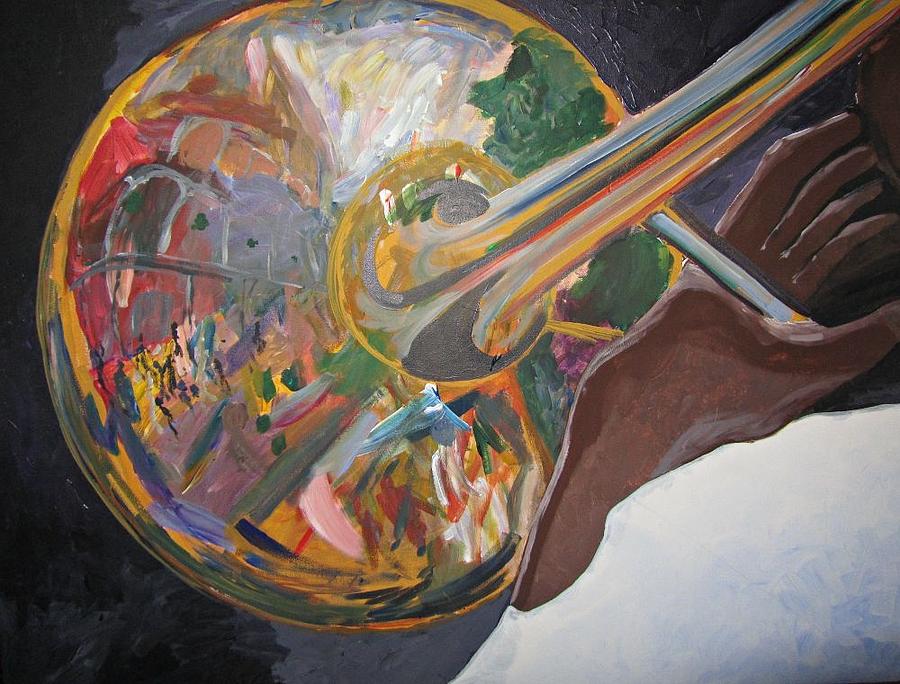This oil painting vividly portrays an African-American trumpet player grasping his trumpet, prominently featuring the colorful, flared bell of the instrument. The bell of the trumpet is depicted with a striking tie-dye effect, showcasing a spectrum of colors including greens, silvers, oranges, purples, blues, yellows, and pinks. The stem of the trumpet extends towards the player's mouth and is similarly adorned with streaks of blue, black, red, yellow, and brown oil paint, adding to the painting's artistic flair. The hand holding the trumpet is rendered in detailed brushstrokes, enhancing the texture and depth of the composition. On the bottom right of the painting, the white canvas is visible with a few blue brush strokes, contrasting with the predominantly black background on the left side, where the brushstrokes are also clearly discernible. This masterpiece blends abstract art with vibrant realism, capturing the dynamic essence of the musical instrument and its player through meticulous and colorful oil brushwork.